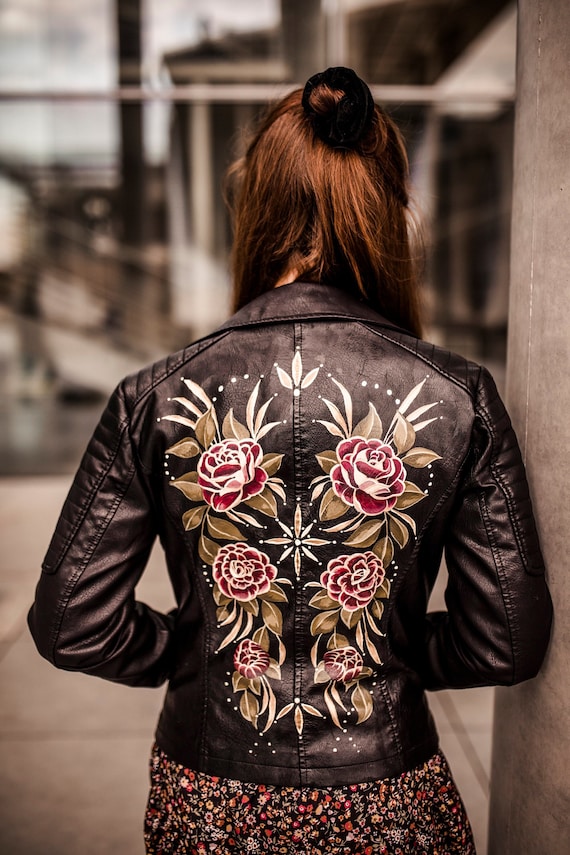In this colored photograph, a woman with red hair is standing outdoors on a sidewalk, her back facing the camera. She wears a waist-length black leather jacket adorned with intricate details. Her hair is tied up in a bun, allowing the entire design on the back of the jacket to be visible. The jacket features six red roses with dark green leaves, arranged symmetrically with three on either side. The roses, which have a delicate white trim on each petal, are connected by light green stems and foliage that climbs towards her shoulders, where the roses appear larger. In the center of the jacket, positioned between the roses, is a beige and white star-like emblem. Below her jacket, she wears a black skirt patterned with multicolored flowers, predominantly yellow and pink. The background of the image is intentionally blurred, offering a hint of reflective windows and possibly a docking area, with a gray wall to the right of the image. The woman stands with her arms pulled in front of her waist, highlighting the detailed seams and decorations on her leather jacket.